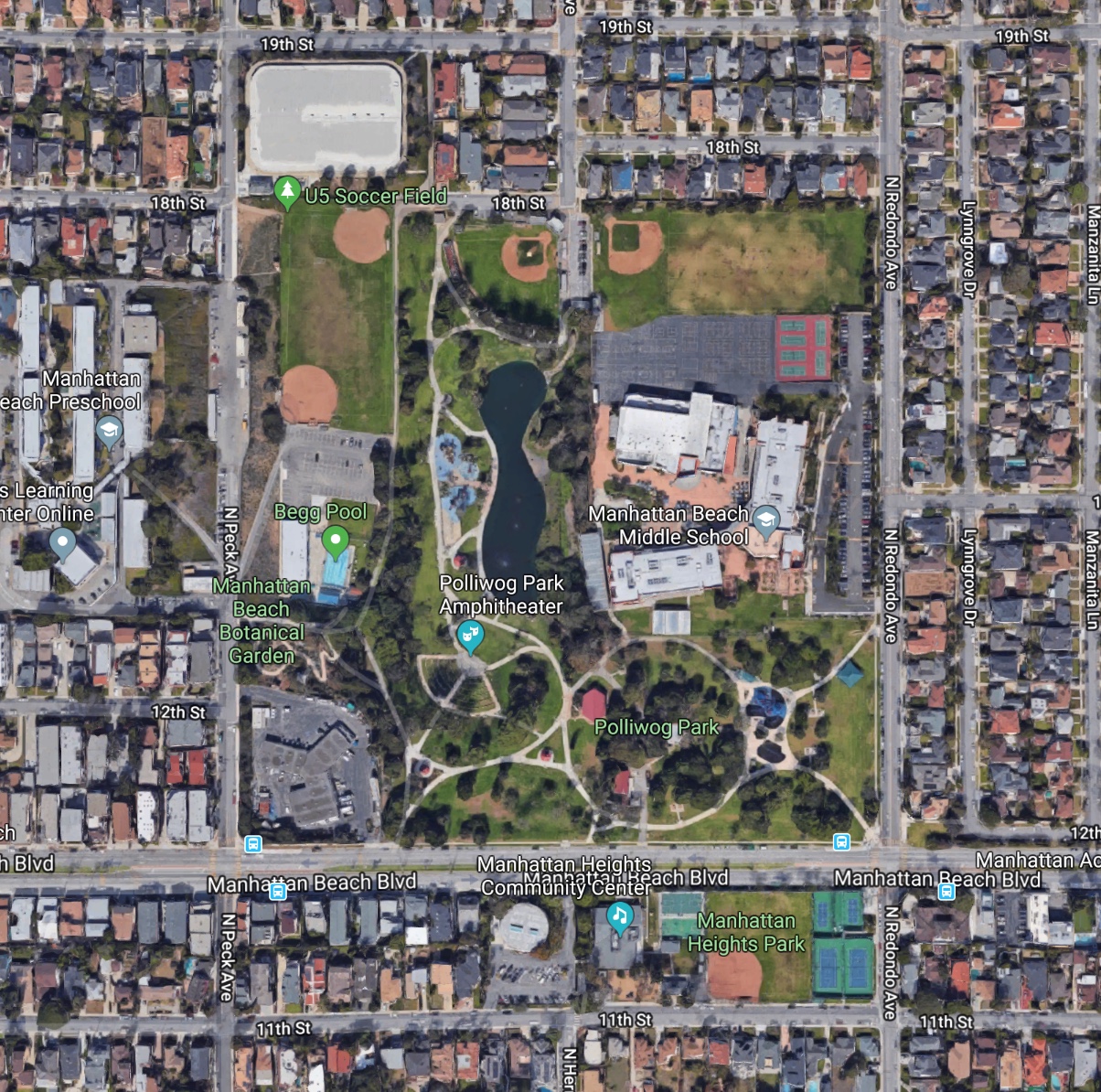This detailed aerial photograph captures a vibrant section of a city centered around a large park that spans five blocks from north to south and four blocks from east to west. In the core of this expansive green space, you will find the Manhattan Beach Middle School, nestled alongside various recreational amenities. An amphitheater is prominently positioned, offering a venue for community events and performances. The park is divided into distinct sections, with a particular area known as Poliwag Park. Nearby, there is a spacious parking lot, a public pool inviting for a swim, and a meticulously maintained soccer field.

Surrounding the park, the modest roofs of residential homes create a picturesque neighborhood. A four-lane street forms a major thoroughfare, while smaller two-way streets provide additional access and connectivity. The image captures the bustling yet serene essence of daytime in this residential area, highlighting the harmonious blend of urban living and natural beauty.